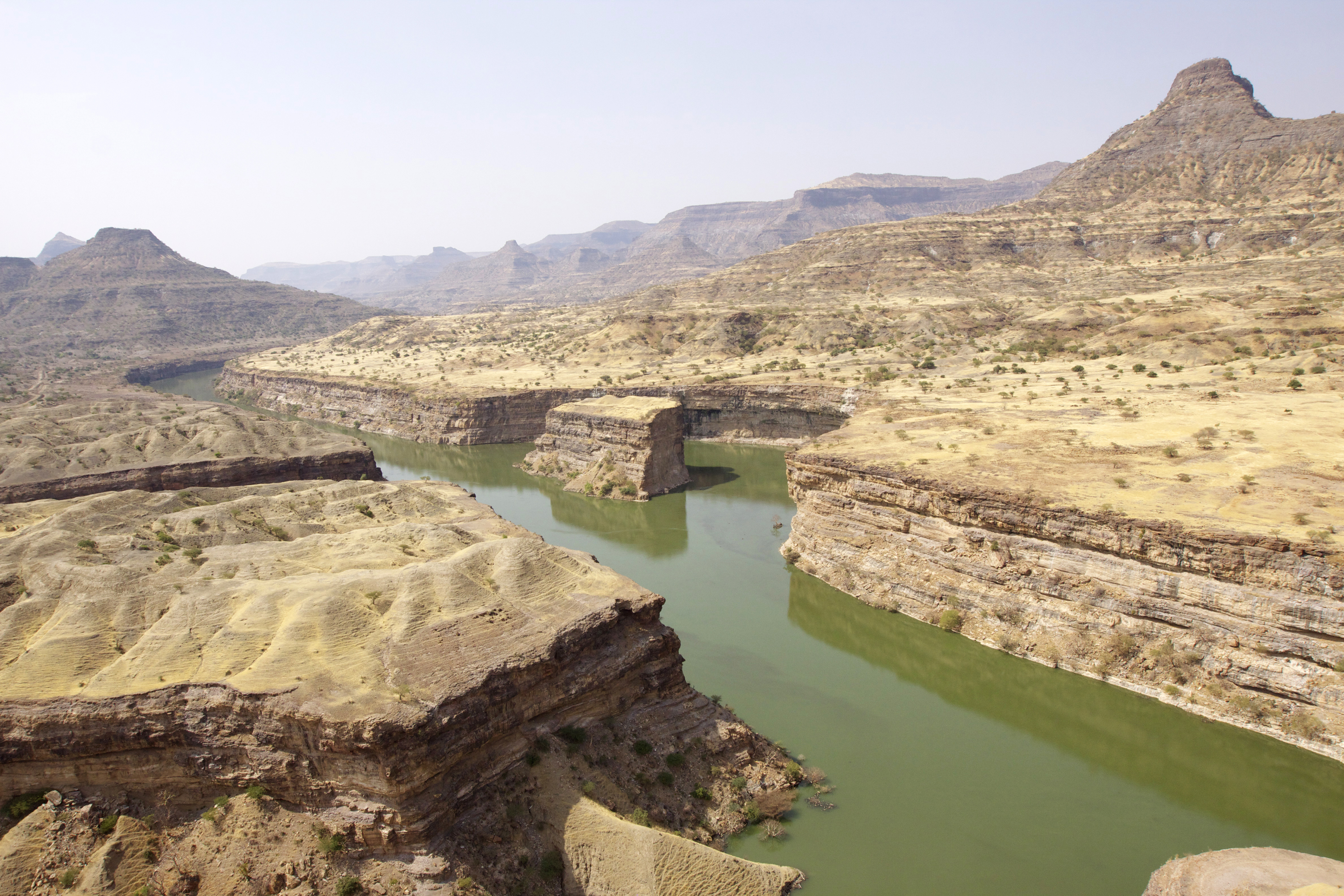This is a color photograph in landscape orientation, capturing an arid, desert-like area from an elevated perspective. The photograph, likely taken from a drone or a high vantage point, looks down towards a canyon that dominates the landscape. The rugged terrain is characterized by rock surfaces and sparse vegetation, predominantly in sand-colored and varying shades of browns and grays. 

Cutting through the barren land is a large creek bed that starts from the bottom right corner of the image and stretches diagonally towards the center-left before curving back to the right and disappearing behind the hills. This water body, colored a murky olive green, appears almost as if it has been carved out of the rock by erosion over time. 

The left bank of the creek features a rocky abutment with a flat top leading down to the waterline through layers of rock, while the right bank has a steep vertical rock wall. An island of rock sits in the center of the creek, with water flow surrounding it. 

In the background, a range of mountains of varying heights rises, with the tallest peak on the right side and a shorter one on the left. The mountains exhibit a grayish-purple hue under a bright, hazy sky that lacks distinguishable clouds, creating a stark and almost surreal contrast against the terrain below. The overall impression is of a hot, dry, and desolate landscape captured in photographic realism.